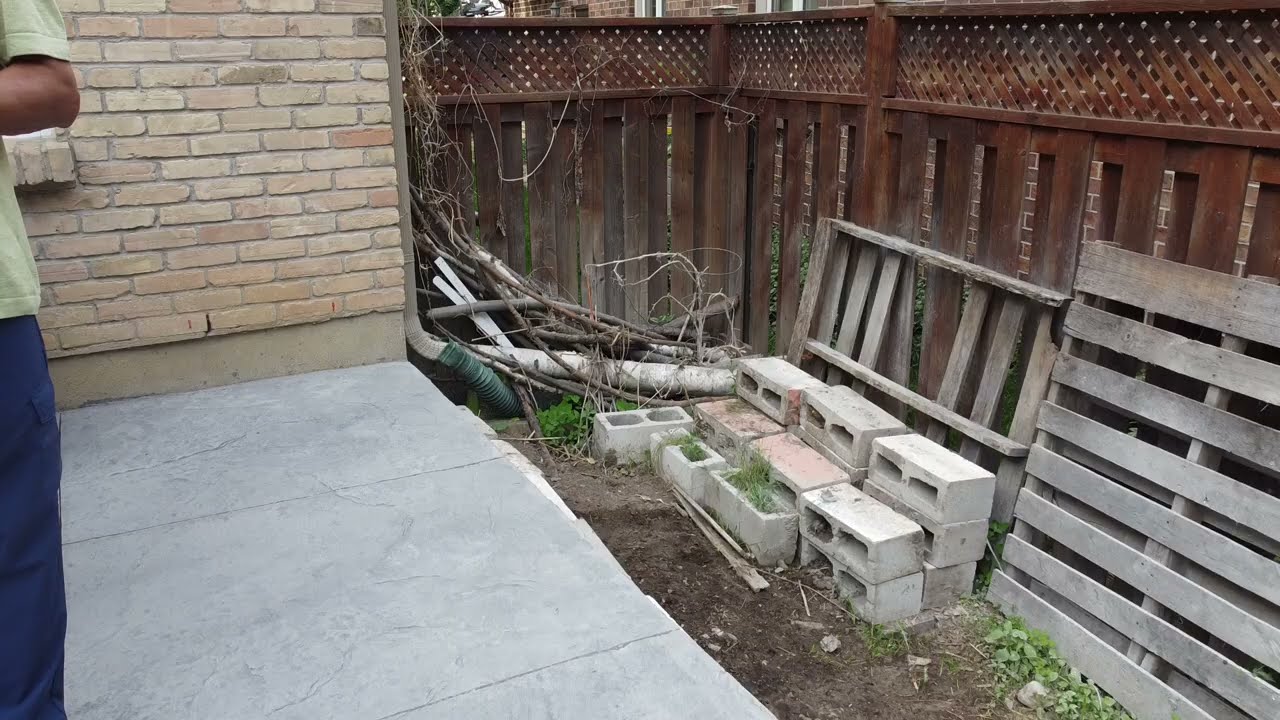The photograph captures a backyard scene with a focus on various construction materials and the surrounding environment. At the center right of the image, there is a structured pile of at least twelve cinder blocks, stacked three rows high. This pile is positioned adjacent to two pallets leaning against a dark wooden fence, which features lattice trim at the top and vertical slats down to the ground. The left pallet appears damaged with missing and broken vertical pieces, while the right pallet remains intact. Beneath and beside the pile of cinder blocks, there are several long gray pavers resting on a cement floor.

To the left, the image shows part of a brick house, with a wall composed of bricks in varying shades of pink and red. A gutter climbs the wall to the right of the house, extending up towards the fence.

Partially visible on the left side of the photograph is a person, identifiable only by their arm and part of their torso. The individual has brown skin and is dressed in blue pants and a light green shirt.

In the background, tangled tree branches and some pipes add to the cluttered scene, along with a hint of moss overgrowing near the fence.